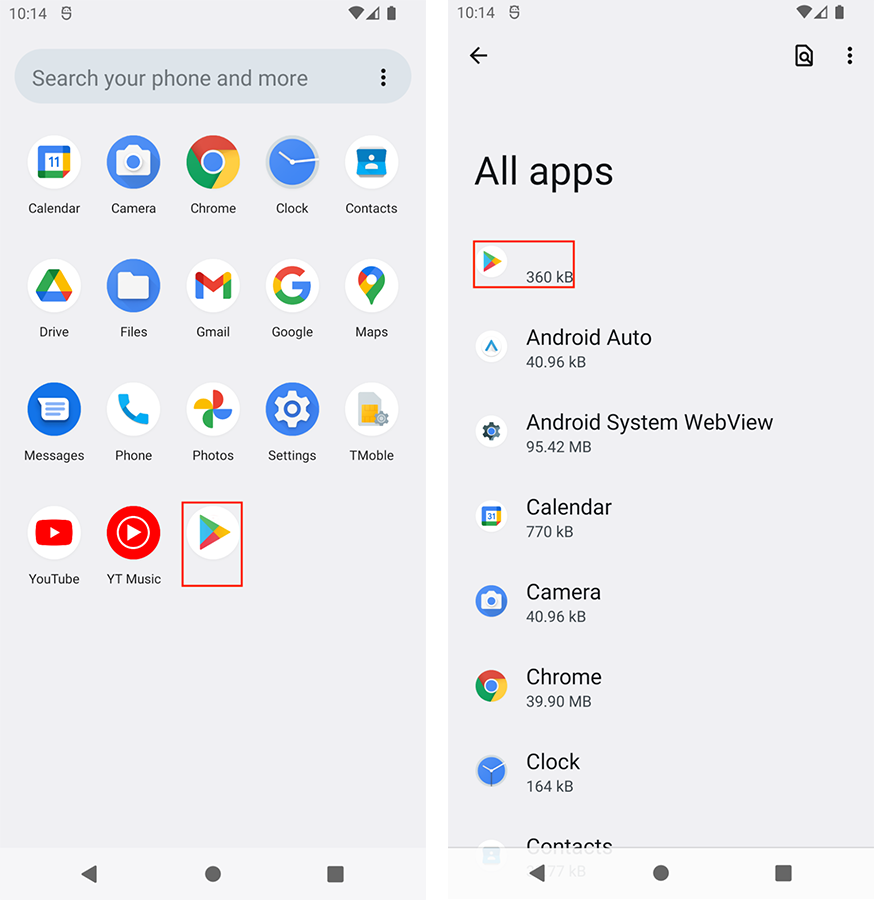The screenshot captures an Android smartphone's home screen, displaying a wealth of information and various app icons. At the top of the screen, an LED shows "1014." The status bar illustrates a fully connected Wi-Fi signal, a battery icon, and a network indicator from T-Mobile. Below, there's a search bar marked by a magnifying glass with the message "search to find more..."

The main interface showcases standard Android shortcuts and functionality icons including:

- Calendar
- Camera
- Chrome Browser
- Clock
- Contacts
- Jive
- Files
- Gmail
- Google Search
- Maps
- Messages
- Phone
- Photos
- Settings
- YouTube
- YouTube Music
- Play Store

Additional app information is available in the "All Apps" section featuring:

- Android Auto: 40.96 kilobytes
- Android System: 5.42 megabytes
- Calendar: 70 kilobytes
- Camera: 40.96 kilobytes
- Chrome: 39.90 megabytes
- Clock: 124 kilobytes
- Contacts

Navigation icons such as a left-facing arrow, a triangle, a circle, and a square appear at the bottom, providing easy access to standard Android operations.